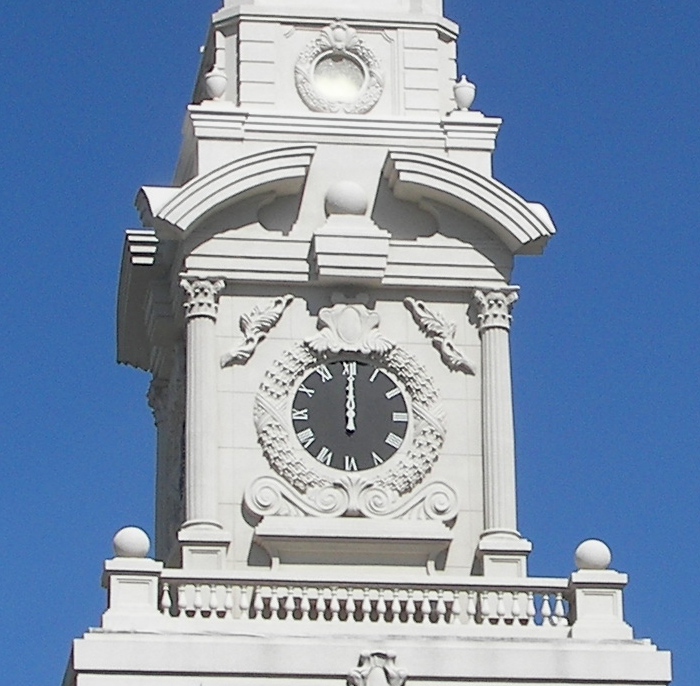The image depicts a towering gray-colored landmark statue featuring a central clock. The base is accentuated by a railing with symmetrical left and right-hand sides, adorned with short, square pillars topped by light gray balls. Rising above the base are two pillars framing a square section that houses a circular clock with white Roman numerals, both clock hands pointing to 12. The design continues upward with curved lines and another gray ball, culminating in a striking blue backdrop flanking the structure.